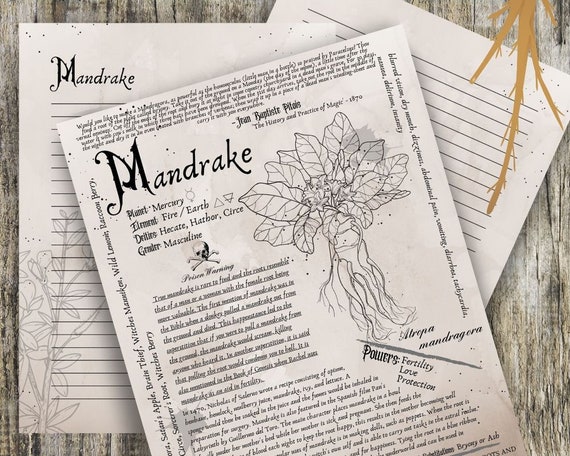This photograph captures a trio of sheets laid out on a grayish-whitish wood surface, primarily revolving around the mandrake plant. The foremost sheet, prominently titled "Mandrake," contains a wealth of information in cursive script, albeit somewhat challenging to decipher. It references astrological elements like Planet Mercury and the elements Fire and Earth, identifying the plant as masculine. A detailed black ink diagram on the right illustrates the mandrake root, complete with a scientific name. Essential attributes such as fertility, love, and protection are highlighted, alongside a conspicuous skull and crossbones symbol indicating poison. The two sheets beneath are less descriptive; the second sheet also sports the title "Mandrake" with faint plant imagery, while the bottom sheet is merely lined paper devoid of additional markings, serving as a subtle backdrop to the primary informative page.